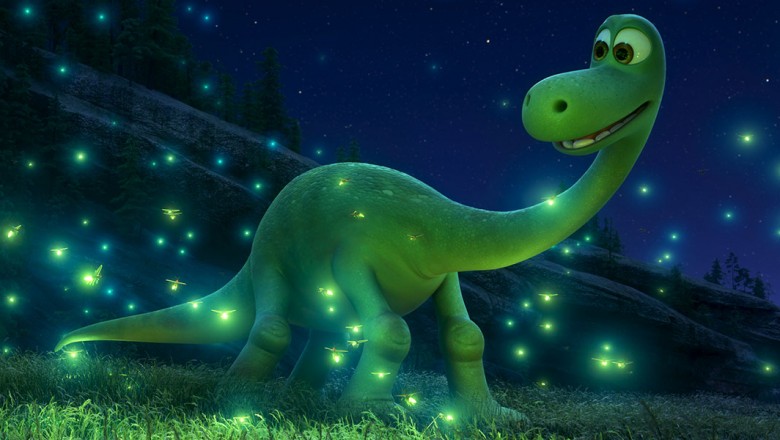In this detailed fantasy drawing, the central figure is a friendly green dinosaur, reminiscent of a brontosaurus, with a long neck, a long tail, and a short body adorned with large kneecaps. Its face, featuring big green eyes, a broad nose with two large nostrils, flat white teeth, and a friendly smile, adds a whimsical charm to the scene. The dinosaur is standing on vibrant green grass illuminated by numerous lightning bugs or fireflies, whose sparkling yellow and green lights create a magical ambiance. The background showcases a deep blue, starry night sky, with faint dark trees visible in the top left corner and a bluish hill adding depth to the scene. The dinosaur, gazing to the left, seems to be interacting playfully with the fireflies that flit around it, casting a warm glow on the grassy ground.